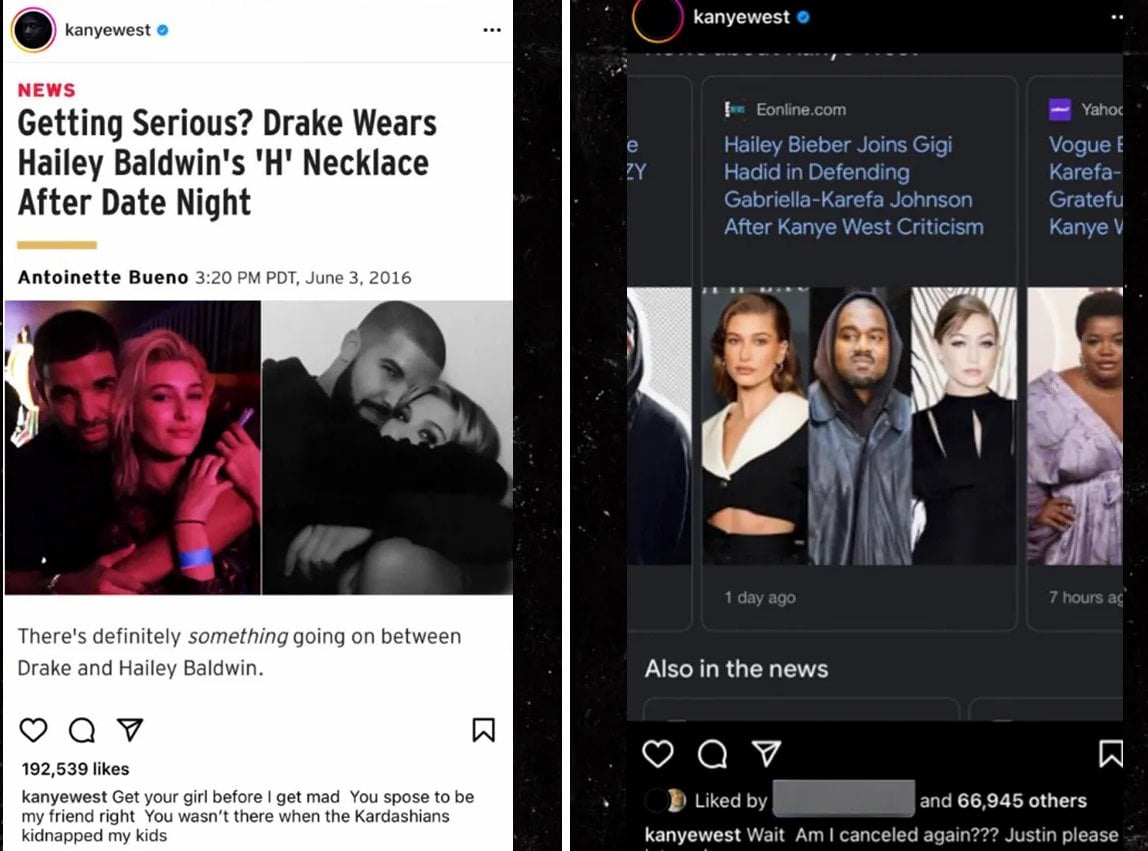Here's a cleaned-up and detailed caption for the image described:

---

This image is a composite of two side-by-side Instagram posts made by Kanye West, both bearing his profile icon, verified blue checkmark, and username.

The post on the left has a white background and is a screenshot of a magazine article with the headline: "Getting serious? Drake wears Hailey Baldwin's 'H' necklace after date night." There are two pictures of Drake and Hailey Baldwin positioned below the headline. The article's caption speculates, "There's definitely something going on between Drake and Hailey Baldwin." This Instagram post has garnered 192,259 likes. Kanye's caption accompanying this post reads: "Get your girl before I get mad. You supposed to be my friend, right? You wasn't there when the Kardashians kidnapped my kids."

The post on the right features a black background and is a screenshot from the Google News section, showcasing an article titled: "Hailey Bieber joins Gigi Hadid in defending Gabriela Carretha Johnson after Kanye West criticism." Below the title, there's a picture of Hailey Bieber, Gigi Hadid, and Gabriela Carretha Johnson. The article itself is not selected, so only the title and picture are visible. This post has received 66,945 likes. Kanye’s caption for this post reads: "Wait, am I cancelled again? Justin, please."

---